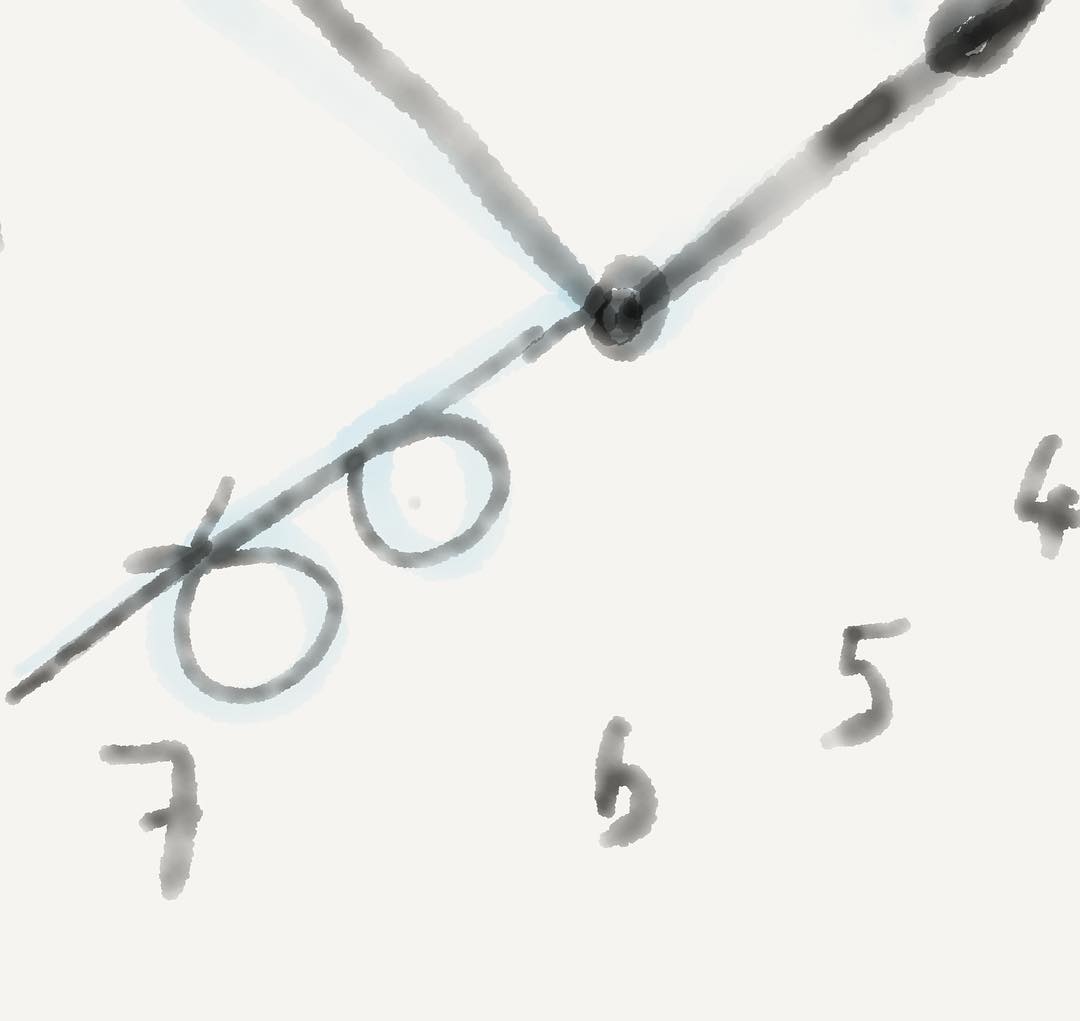This hand-drawn illustration, created with light gray ink and watercolor on a white background, depicts a partial clock face. From the right center bottom, the numbers four, five, six, and seven are arranged in a descending circular pattern. At the clock's center are the hands: the hour hand points toward the upper right corner, the minute hand extends to the top left, and the second hand is angled toward the bottom left. Adding an artistic touch, a few circles are drawn beneath the second hand in the same grayish watercolor, complementing the overall delicate and ethereal aesthetic of the piece.